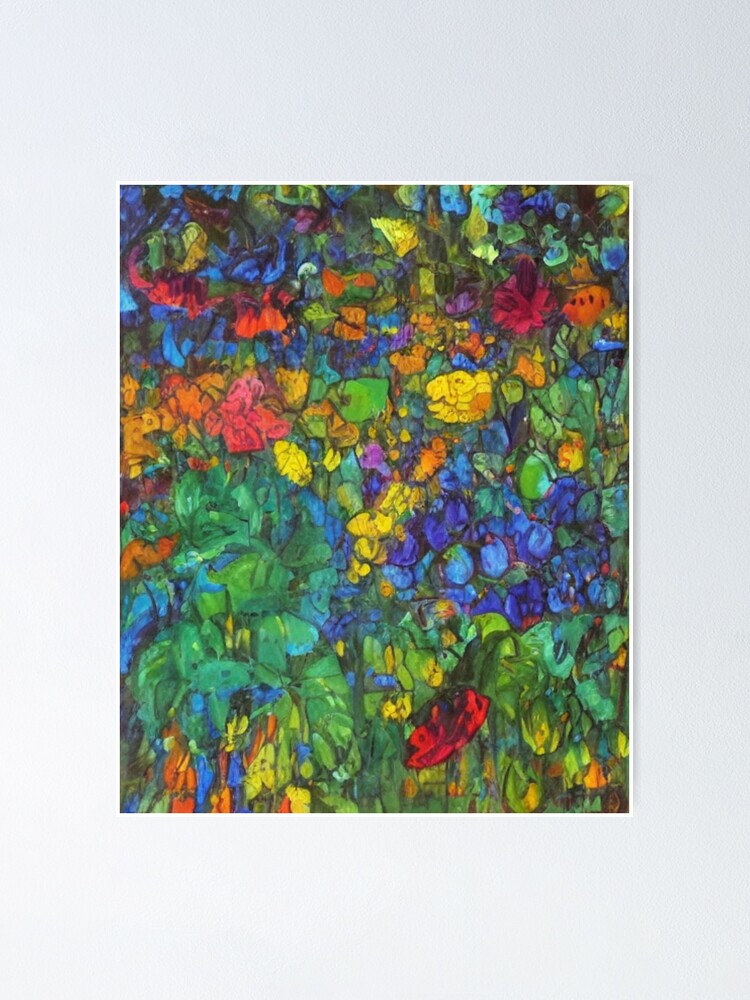The image is a detailed print of an abstract painting with a thin, wide border framing the composition. The background is primarily blue, incorporating both lighter and darker shades. The piece is a vivid explosion of colors, including prominent yellows, greens, oranges, reds, blues, and purples. These colors intermingle in a chaotic yet captivating manner, characterized by irregular, squished oval shapes and amorphous forms that overlap and merge into one another.

The painting seems to depict an array of flowers and leaves, but the forms are so distorted and clustered that they become difficult to distinctly identify. Patches of green dominate the background, populated by various clusters of flowers in contrasting colors. Notably, there is a bright red flower at the bottom right, blue grape-like flowers above it, and an assortment of yellow, orange, and red blooms higher up in the composition. The overall effect is a muddled but richly colorful tapestry, conveying the sense of floral abundance without clear definition.